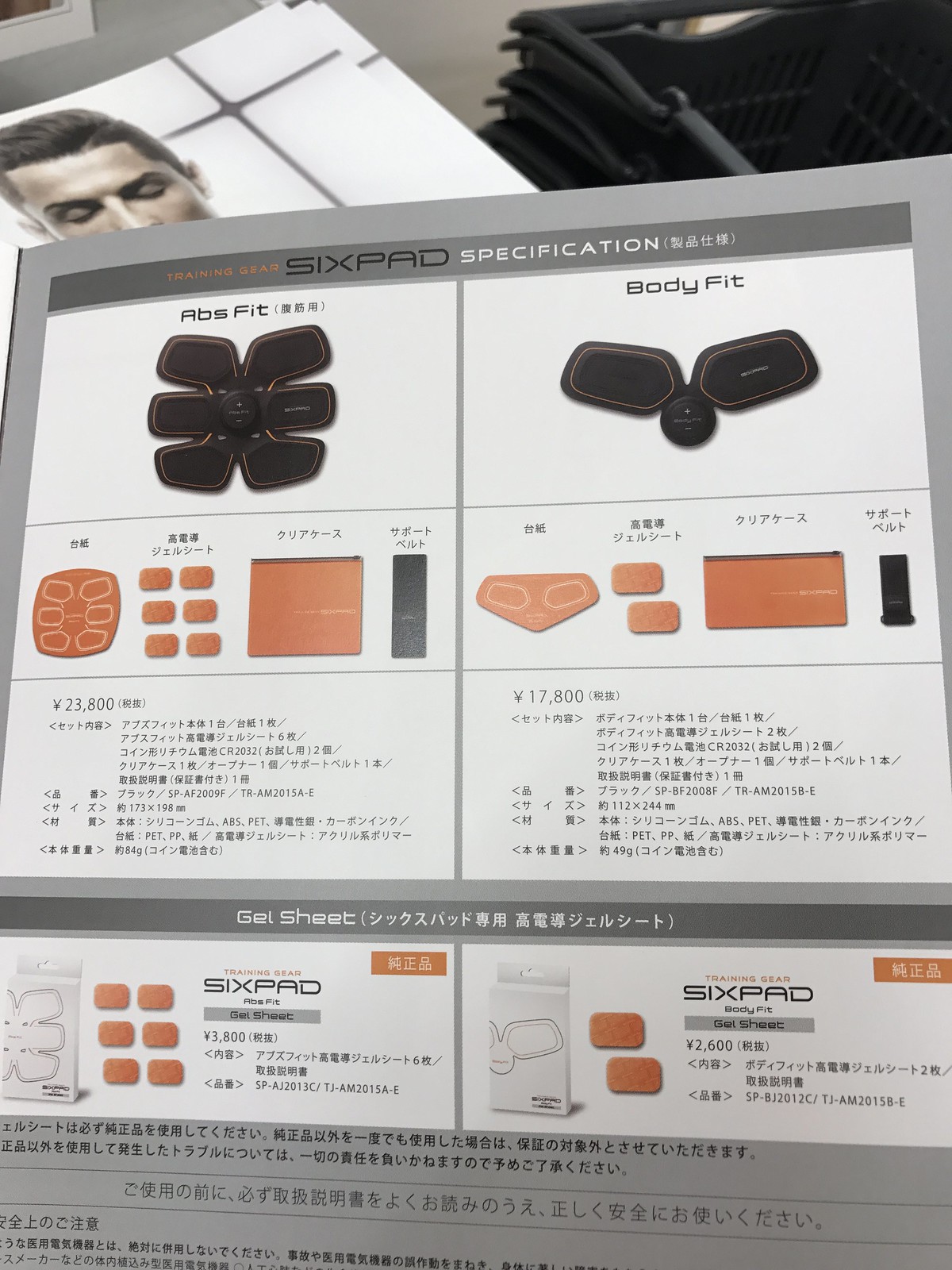The image is a Japanese catalogue advert for a body training tool that utilizes electrical muscle stimulation pads. These pads, available in two versions – AbsFit and BodyFit – are designed to adhere to the body's abdominal area for exercise purposes. The AbsFit is priced at ¥23,800, while the BodyFit is offered at ¥17,800. Detailed instructions and pricing are provided in the advert, which predominantly features shades of gray, white, and peach-orange. The background of the advertisement includes an image of a male with dark hair who resembles Ronaldo, looking down, possibly with his eyes closed. The device itself is black and compact, featuring multiple black adhesive tabs that attach to the skin for effective muscle stimulation.